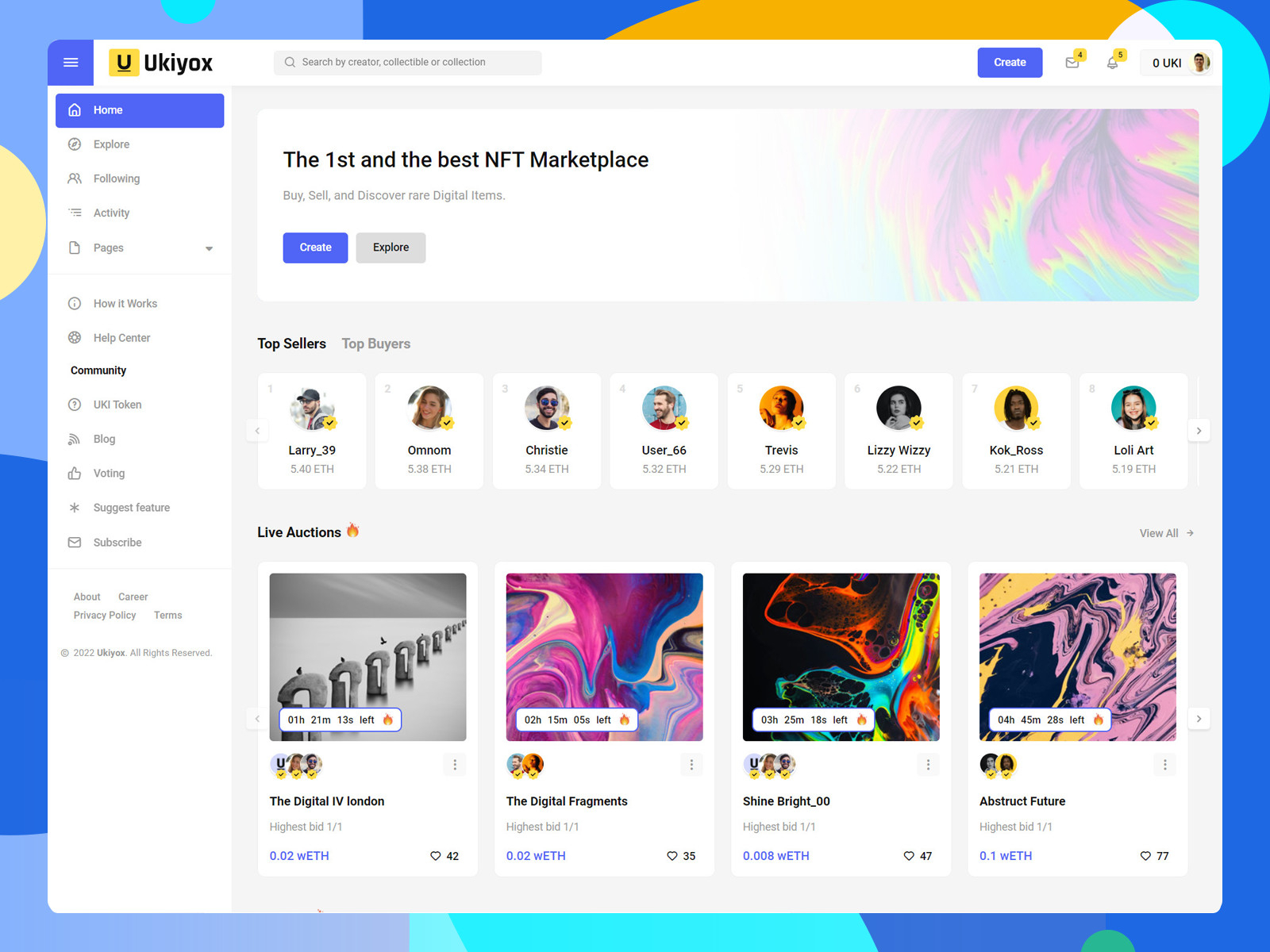The image features a bordered interface with a color scheme composed of dark blue, orange, light blue, tan, teal, and a combination of dark green and light green. Inside the border is a central menu or page displaying the text "UKLYOX," adjacent to a yellow box. Directly below this, a dropdown menu is positioned, reading "The first and the best NFT marketplace. Buy, sell, and discover rare digital items." 

To the right of the dropdown menu, there are two buttons: one blue button labeled "Create" and one gray button labeled "Explore." Beneath this section, the interface highlights categories labeled "Top Sellers" and "Top Buyers." This area features eight white squares, each containing a profile picture and a corresponding username. The listed usernames include: Larry_39, OMNOM, Christy, User_66, Travis, Lizzy Wizzy, and Cock Ross.